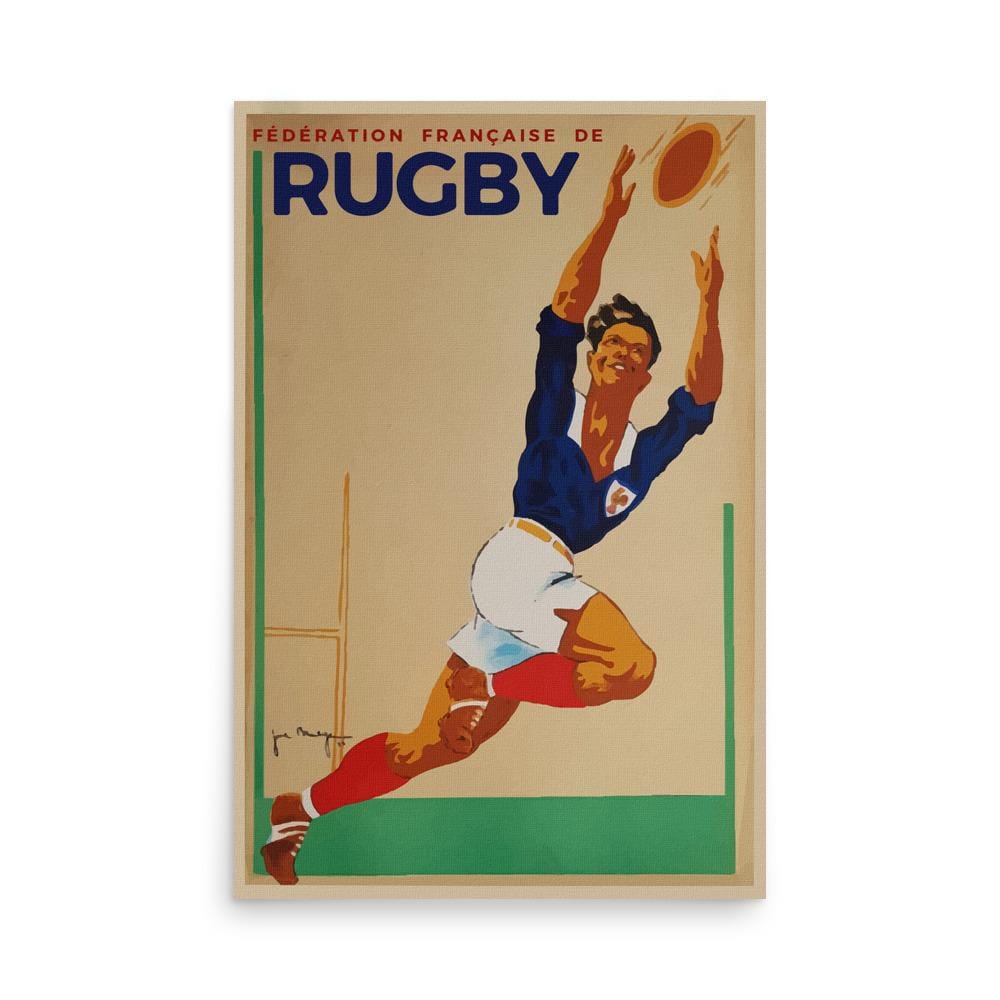The image depicts an old French rugby program cover featuring an artist's rendition of a rugby player. It has a yellowed background, possibly due to age, with a green indent and a green border along the bottom. At the top, in red text, it reads "Fédération Française de Rugby." Dominating the cover is a cartoonish depiction of a rugby player with black hair blowing in the wind, outfitted in a blue jersey with rolled-up sleeves, white shorts secured with a tan belt, and red socks paired with brown cleats that have white laces. The player is captured in a dynamic pose, with arms outstretched as if to catch a ball—an orange, disc-like object with yellowish accents. His left foot is firmly on the ground while his right foot is bent upwards, mid-stride. To the left of the player, a goal post and a black script signature are visible. The background also includes blue lettering spelling out "rugby," adding a pop of color and emphasis to the magazine-style cover.